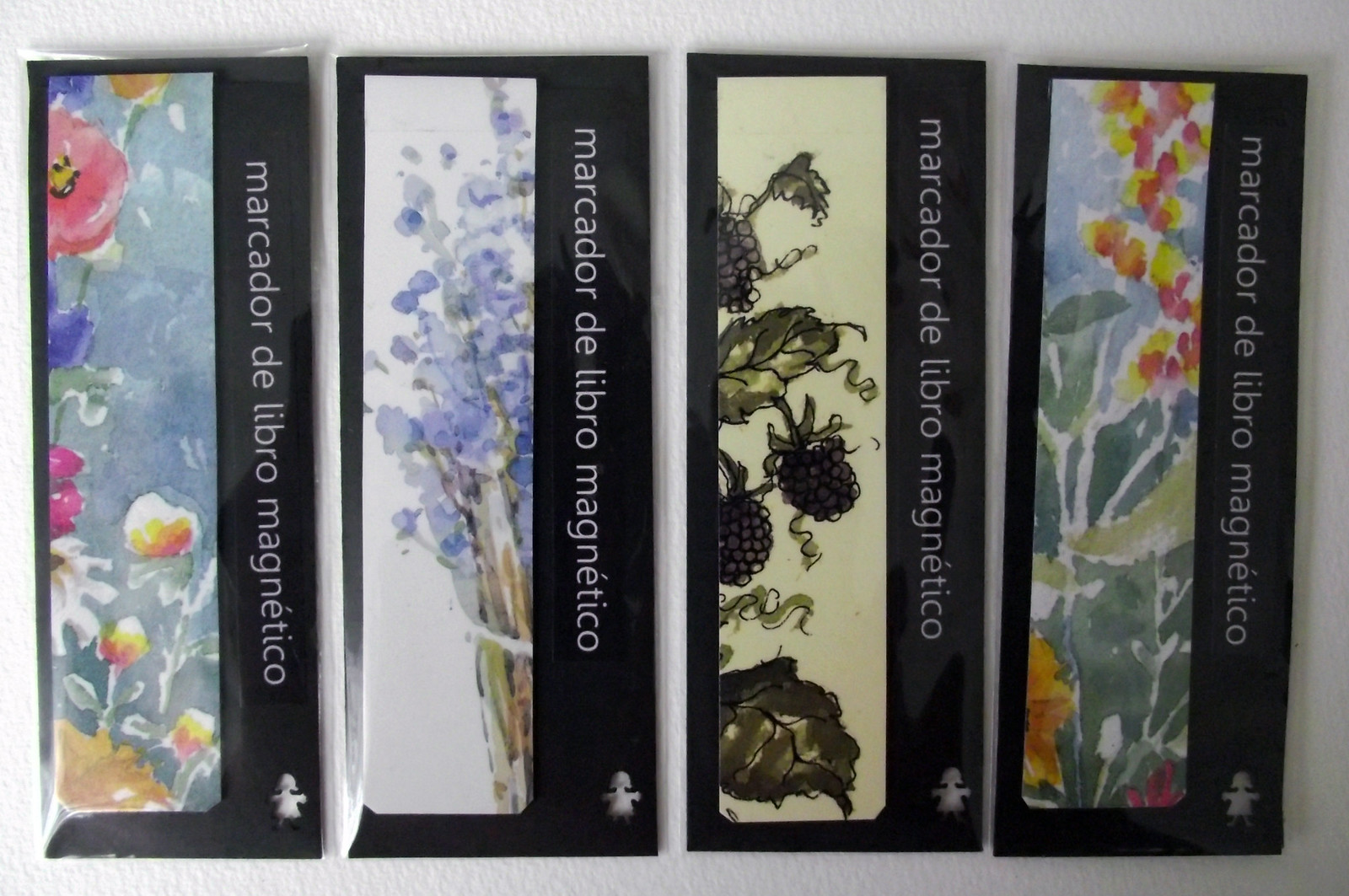In this photograph, there are four rectangular packages arranged side by side, neatly stacked in a line. Each package features a black border with thicker sections on the right side and the bottom, and a thinner trim on the top and left sides. The main section of each package is occupied by whimsical watercolor illustrations depicting various flowers and vegetation, exuding a fanciful, nature-inspired charm. Vertical text in gray lettering, "Marcador de Libro Magnetico," runs down the right side of each package, indicating that these are magnetic bookmarks. At the lower right corner of each bookmark, there appears to be a small, possibly child-like or scarecrow stick figure. The text suggests a Spanish context, further affirming their purpose as magnetic page markers. Despite some confusion about their potential multipurpose use, these beautifully illustrated and thoughtfully designed items are clearly intended to serve as bookmarks.